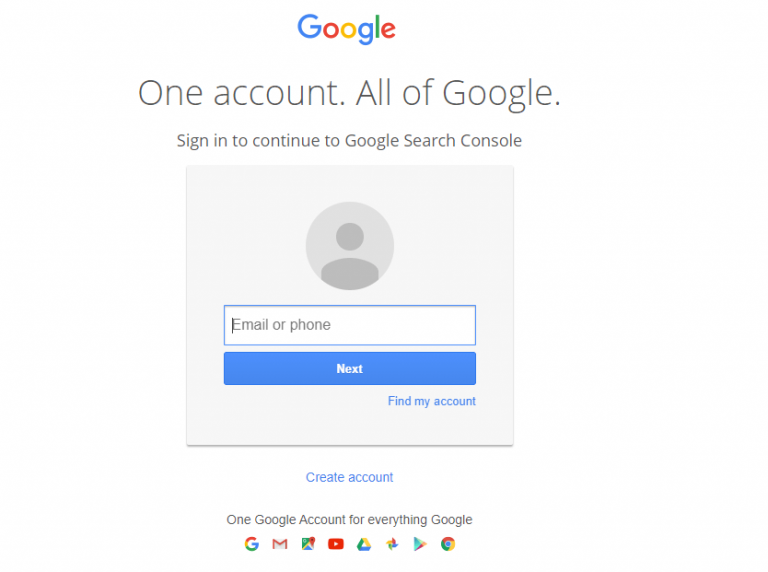This image is a screenshot of a Google login webpage with a clean white background. At the very top center, the colorful Google logo is prominently displayed, showcasing the word "Google" in its signature multi-primary colors. Directly below the logo, in large gray font, the text reads "One account. All of Google." Below this, there is smaller font text that states, "Sign in to continue to Google Search Console."

Further down, a light gray square contains a darker gray circle at the top, which features a silhouette of a person in an even darker gray shade. Below the circle, a white input box outlined in blue invites the user to type in their credentials, displaying the placeholder text "Email or phone" in gray font. Beneath the input box, a blue button with white text reads "Next." Below this button, there's a blue text link that says "Find my account."

Underneath the gray square, there’s a smaller white bar with blue font that says "Create account." Following this is a line of black text that declares, "One Google account for everything Google."

At the very bottom of the screenshot, several iconic Google service icons are displayed. These include the icons for Google, Gmail, Google Maps, YouTube, Google Docs, and Chrome, representing the array of services accessible with a single Google account.